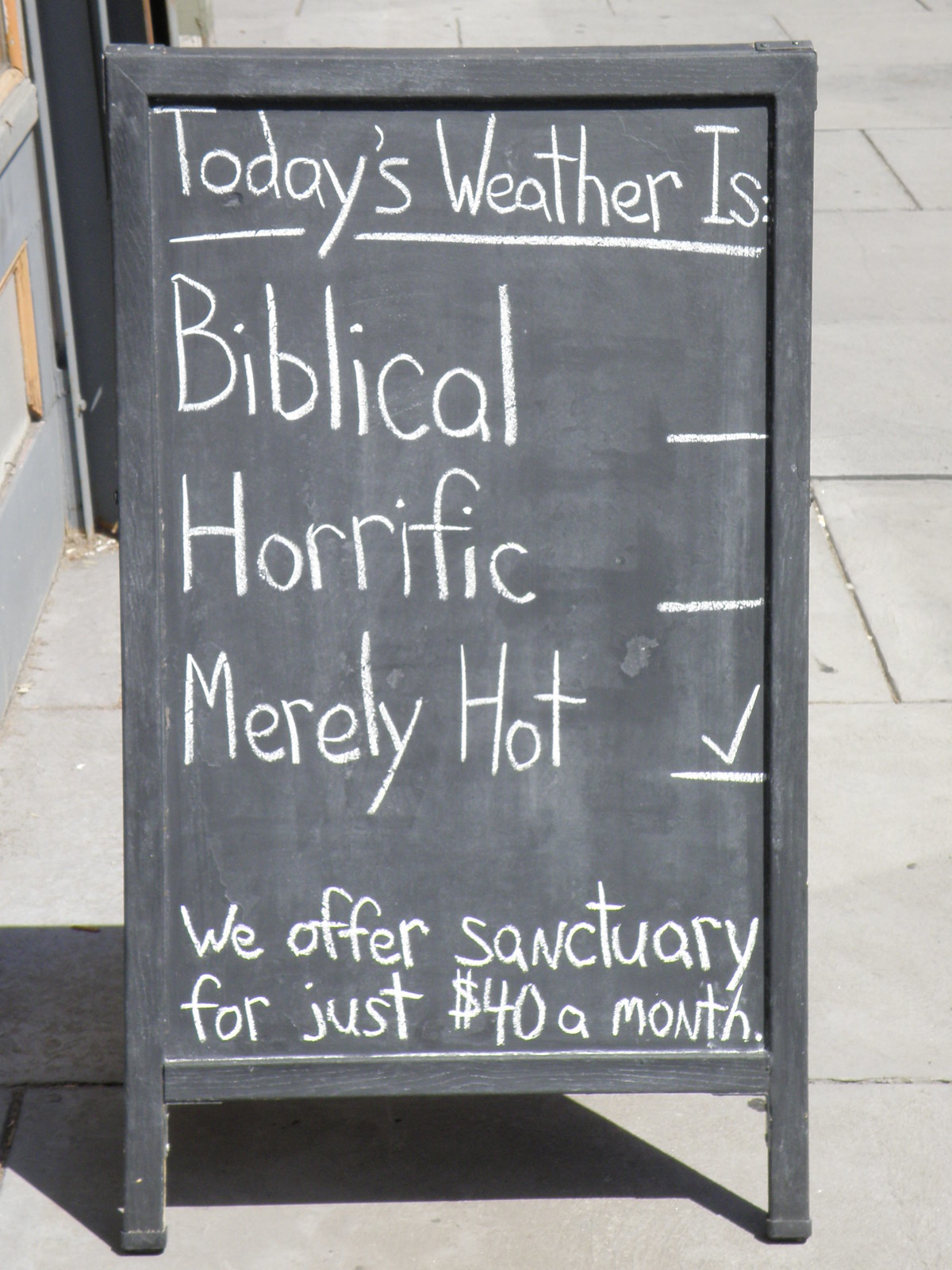The photograph captures an outdoor scene featuring a black A-frame chalkboard sign placed on a gray sidewalk surrounded by concrete bricks. The sign, standing in an easel, bears a shadow cast to the bottom right, indicating it’s daytime with the sun primarily in front of it. The chalkboard displays handwritten white chalk lettering that reads:

"Today's weather is:"

This is followed by three vertically-listed categories:
1. "Biblical" 
2. "Horrific" 
3. "Merely Hot" with a checkmark next to it.

Further down, the sign advertises, "We offer a sanctuary for just forty dollars a month."

In the background to the left of the sign, there’s a glimpse of a gray doorway leading into a building, contributing to the urban feel of the setting while the remaining background is dominated by the sidewalk and part of the building structure, leaving the focus on the chalkboard's quirky weather update and offer.